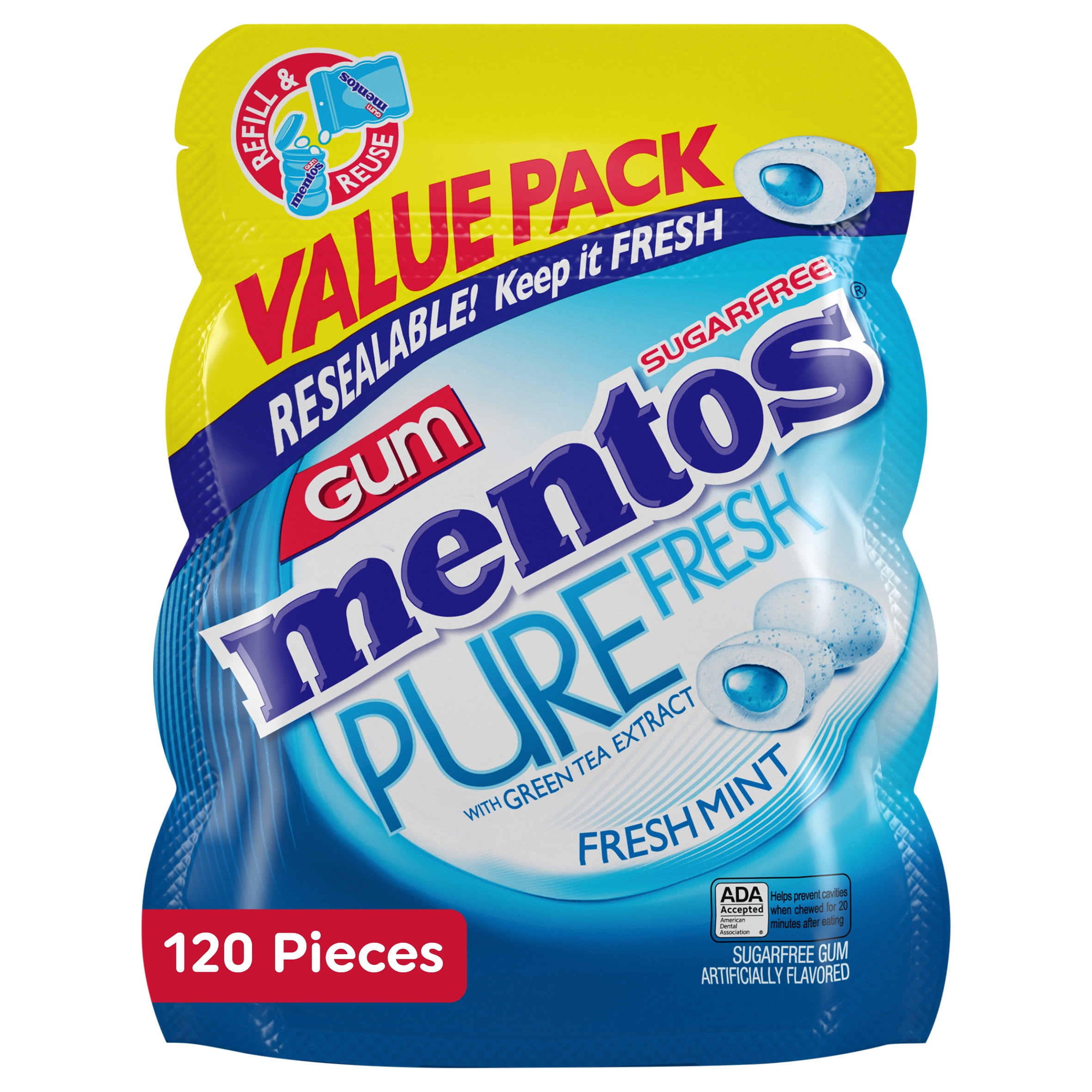This is a detailed close-up image of a value pack of Mentos gum. The packaging is designed to be torn open for easy access. At the top, the words "Value Pack" are prominently displayed in red lettering on a yellow background. Below this, the text "Refill and Reuse" indicates that the gum can be poured into one of Mentos' plastic containers for their Pure Fresh line, exemplified by an illustration showing the process. 

The bottom section of the packaging features a blue background with white accents. Here, the product name is clearly visible: "Mentos Sugar-Free Pure Fresh" with the additional note "with Green Tea Extract" beneath. The flavor, "Fresh Mint," is also specified. The package includes images of the gum pieces: one whole piece and two halves that reveal the liquid-filled interior, highlighting the gum's unique texture and composition.

On the bottom-left corner, a red rectangle prominently displays the text, "120 Pieces, Sugar-Free Gum, Artificially Flavored," indicating the quantity and nature of the product. This pack ensures a substantial supply of Mentos gum perfect for those who appreciate long-lasting freshness.